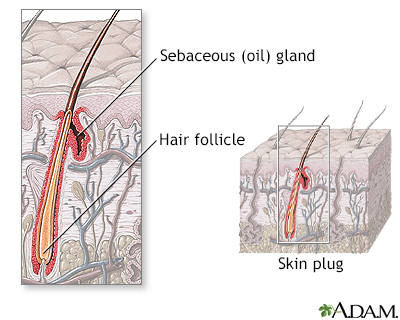This detailed anatomical illustration, likely from an educational pamphlet or book, depicts a skin plug with an emphasis on the structure of a hair follicle in a sebaceous oil gland beneath the skin's surface. Presented in grayscale, the diagram features a side view and close-up of the hair follicle's intricate parts, highlighted with distinctive colors—red on the outer layer and yellow on the inner layer. The images appear hand-drawn, with a larger overview image and a smaller, identical inset for enhanced detail. Notable elements include a sebaceous oil gland depicted in bright red, and a green plant-themed logo labeled "A.D.A.M." on the diagram, suggesting a potential acronym. The diagram also provides an enlarged cross-section of a cube indicating the irritated follicle distinguished from the surrounding follicles.